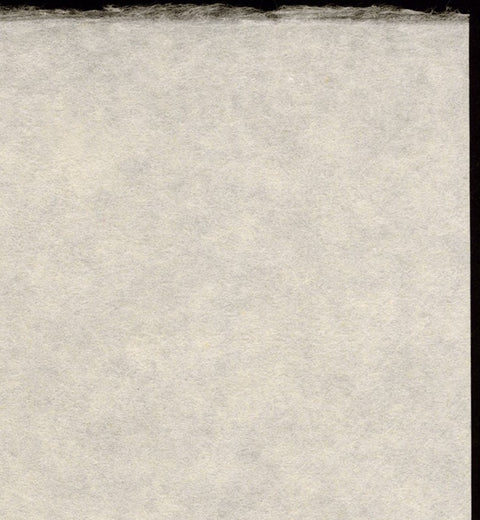The image appears to be a photograph of a vertically rectangular object, possibly an air conditioner filter or a piece of textured material such as paper or fabric. The central focus of the image is filled with a white, cottony or papery surface that exhibits subtle variations in color, including shades of white, light gray, and very pale purple. Towards the top, the material looks slightly fuzzy or hairy, suggesting it might be torn or frayed. To the right, there's a small black border running from top to bottom, providing a stark contrast to the predominantly white surface. The overall texture is intricate, with no symbols or markings, creating a blank, yet richly detailed canvas against a definitive backdrop.